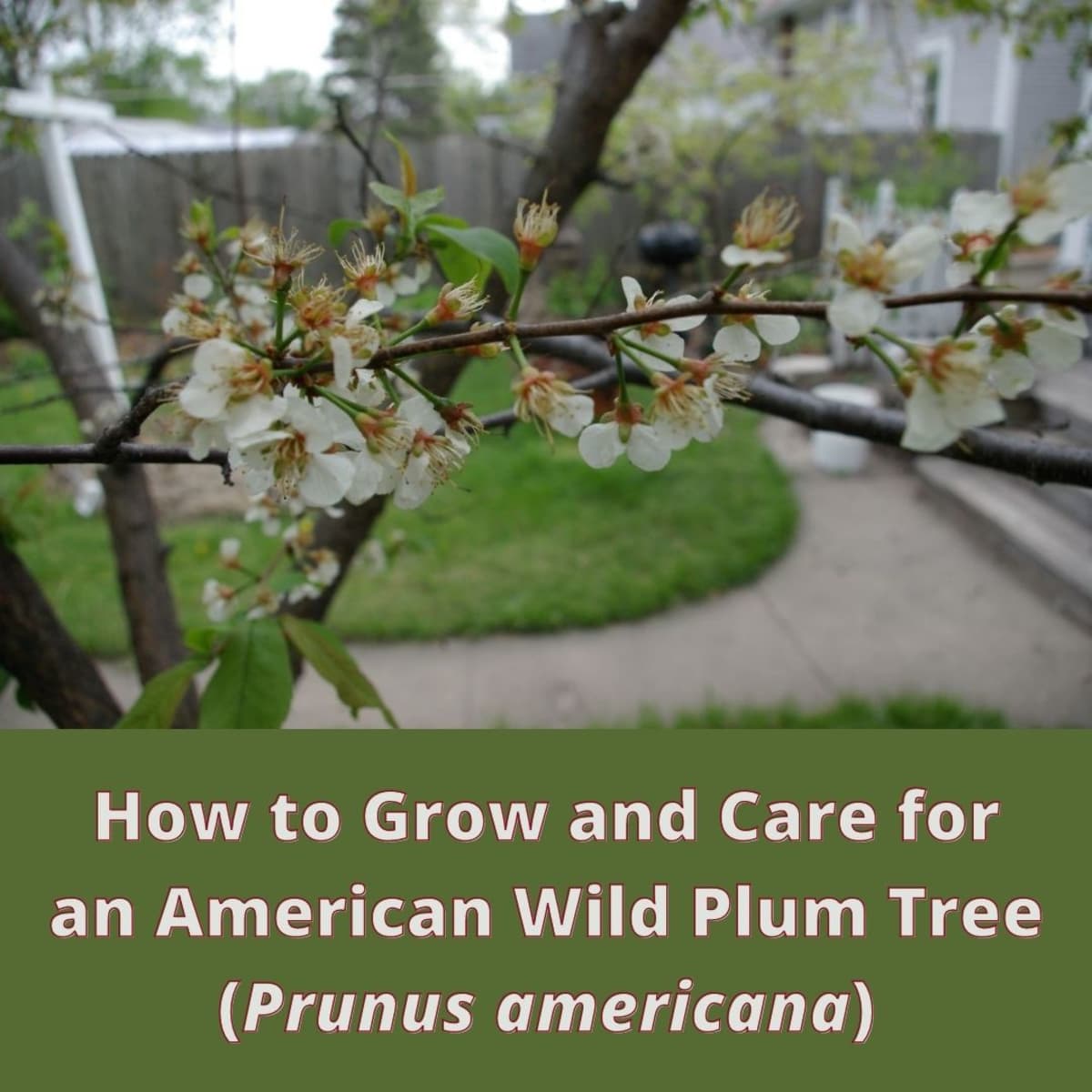The front page of this plant care guide showcases a close-up photograph of a small, thin branch adorned with white plum petals and emerging green leaves, likely from an American wild plum tree (Prunus americana). The vivid foreground highlights the delicate blossoms and slender stems, providing a detailed view of the tree’s flowering stage. Below the photograph, the bottom third of the image features a green field with the text, "How to Grow and Care for an American Wild Plum Tree" and its scientific name in parentheses. In the slightly blurred background, the scene depicts a typical American suburban backyard with a brown wooden fence, a small black grill, and hints of neighboring houses, suggesting a domestic setting. Additional elements such as a concrete walkway, steps leading to a home, and a signpost enhance the suburban atmosphere of the image.